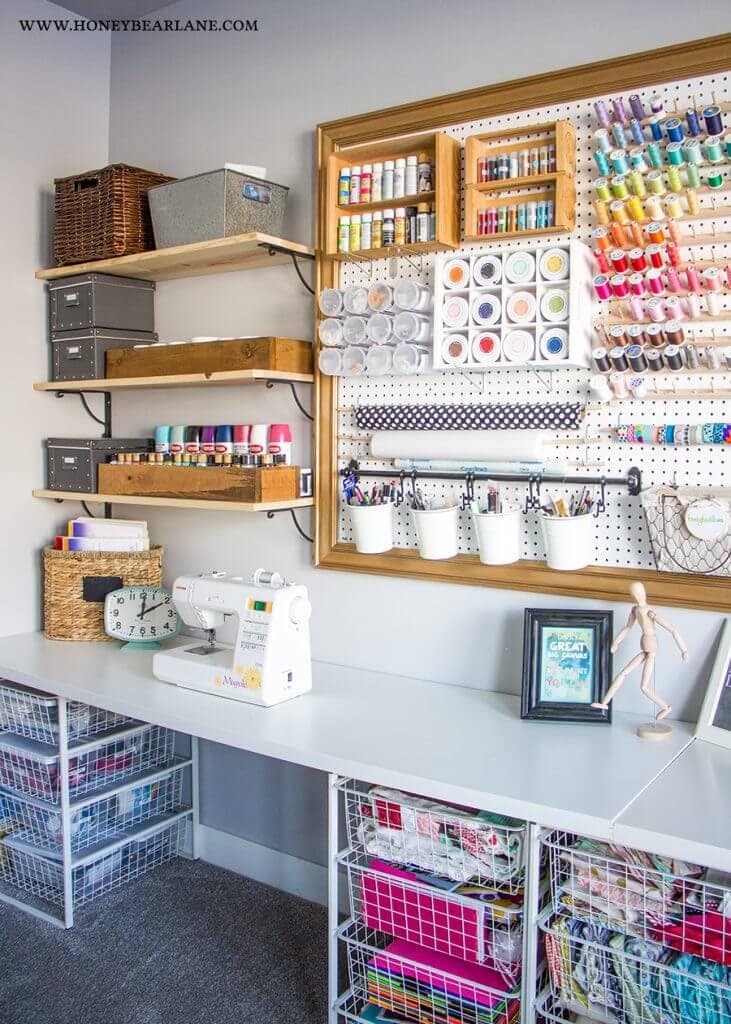This detailed photograph captures one wall of a vibrant craft room, bathed in daylight and showcasing an array of artistic supplies and tools. Mounted on the left section of the white wall are a series of shelves holding various small boxes, cases, and jars filled with crafting materials like paints. A recognizable feature is the white pegboard on the right, designed with a grid pattern of holes to attach pegs and shelves. This board is adorned with an upright metal stand displaying a rainbow spectrum of thread spools, where colors transition from purple at the top, down through blue, green, yellow, red, and pink. Nestled among these are buckets containing colored pens, paintbrushes, and other artistic tools. 

On the counter, which sports a functional white shelf at its base, sits a white sewing machine accompanied by a light blue-faced clock and a weave basket filled with books. An adjustable wooden stick figure, typically used for drawing or painting reference, stands nearby. Underneath the counter, white wire baskets are arranged, brimming with a diverse assortment of colorful paper, fabric, and linens. Additionally, there are visible tubes and cans of materials organized neatly, reinforcing the craft-focused ambiance of the space. The cohesive setup indicates a workspace dedicated to sewing and various forms of artwork, reflecting creativity and meticulous organization.